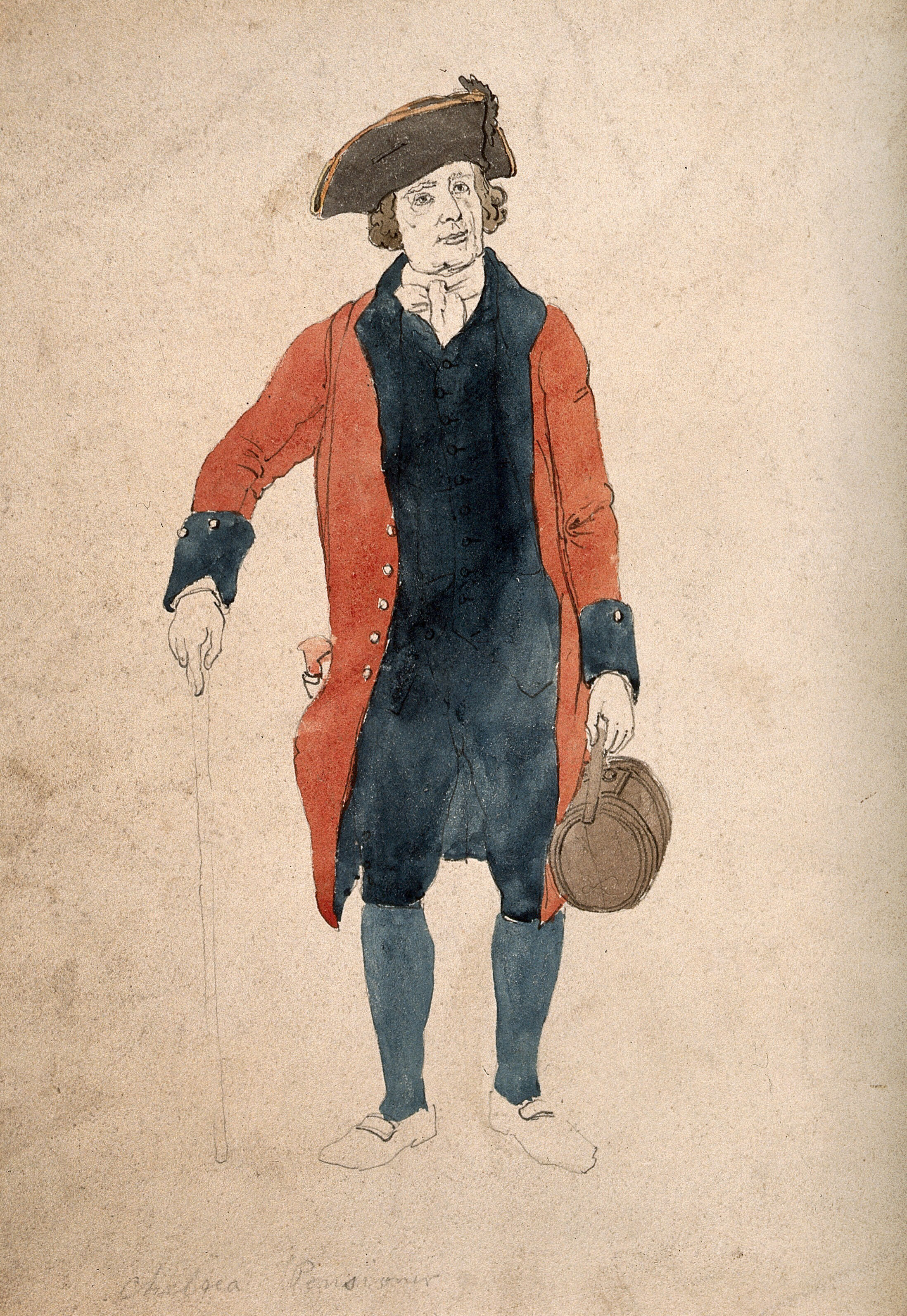The image is a detailed, hand-drawn sketch or portrait, possibly of a historical figure from the 1700s, done in pen and ink and filled in with watercolor on a brownish-beige parchment-like background. There is nothing in the background, emphasizing the figure. The character, who appears to be dressed in a Meneghino costume—a traditional outfit often associated with colonial or Pilgrim periods—features prominently in the artwork. He is wearing a distinctive tri-corner hat and a long red coat with blue trim around the sleeves. Underneath, he has a black vest, a white shirt tied at the neck, green stockings, and bloomer-like pants. He is holding a wooden cane or hiking stick in his right hand. In his left hand, he carries a rounded, brown satchel with a leather strap. The figure is looking off to his left, our right, with some of his hair visible below the hat. While the painting is incomplete, showing unpainted outlines, the detailed depiction suggests a colonial-era European, possibly French, persona, adding historical depth to the portrayal.